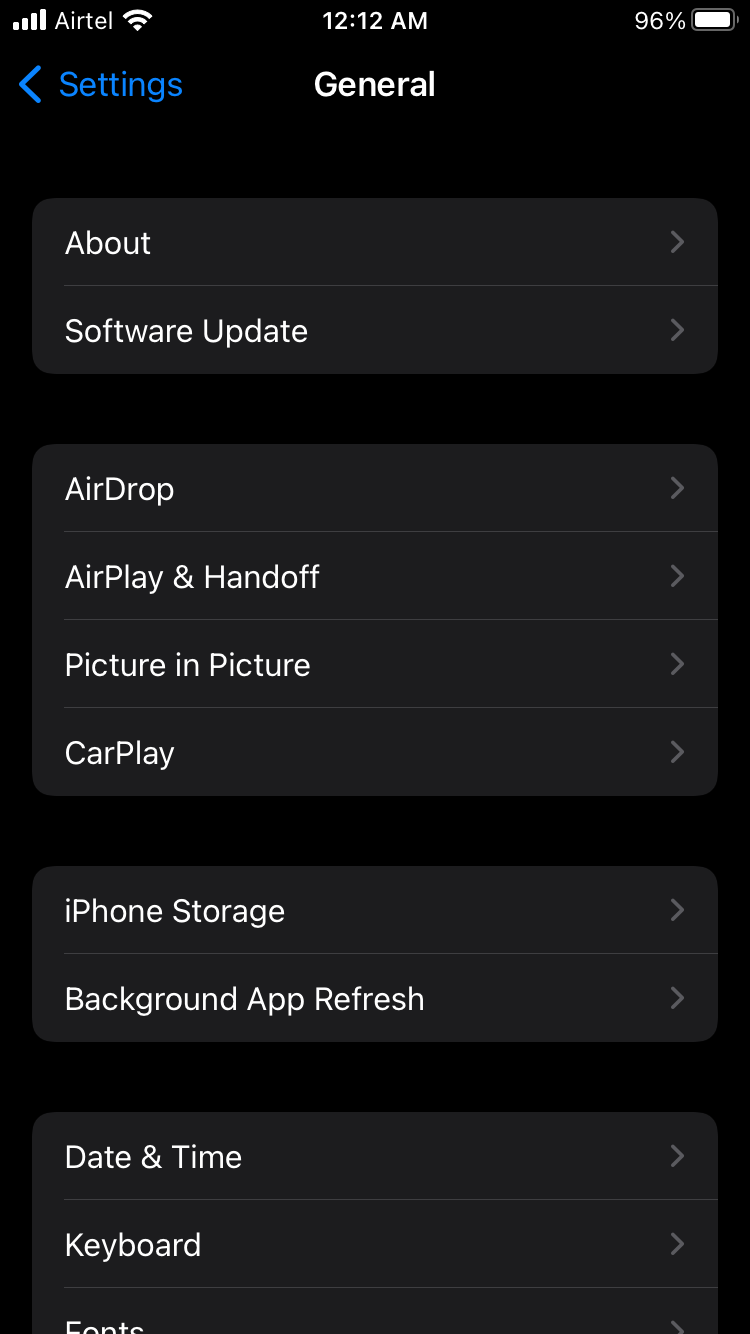This vertically oriented screenshot captures the General Settings menu on an iPhone. At the top-left corner, "Airtel" appears next to four vertical signal bars, indicating network strength, accompanied by a small icon. The current time, "12:12 AM," is centered at the top, while the battery icon on the top right shows a 96% charge. Below these indicators, the screen shows the header "Settings" in blue text with a left-pointing arrow, followed by the word "General" to indicate the current submenu. The backdrop is jet black, emphasizing the interface elements.

The settings options are displayed in long, gray horizontal boxes with a scroll bar on the right. The sections listed from top to bottom are: About, Software Update, AirDrop, AirPlay & Handoff, Picture in Picture, CarPlay, iPhone Storage, Background App Refresh, Date & Time, Keyboard, and Fonts. All the text except for the "Settings" header is in white. The image details strongly suggest it was captured with almost a full battery charge.